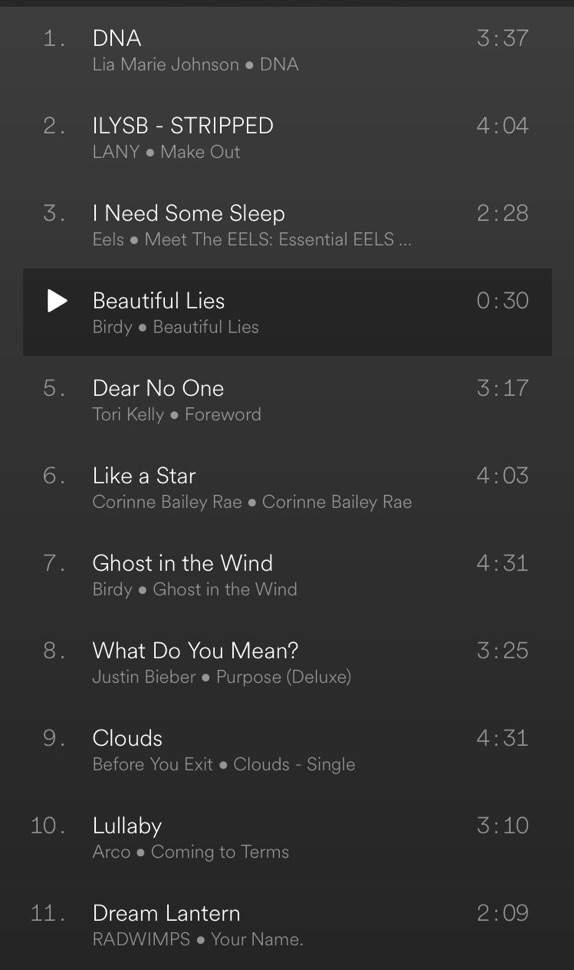The image shows a vertically oriented rectangular list containing 11 items, each denoted with a number except for one which features a play button. The list is characterized by a mix of fonts in white and gray on a slate gray background, except for one entry which stands out with a sharp black background. Here's the detailed breakdown of the items:

1. "DNA" by LaMaria Johnson, "DNA" – 3:37
2. "ILYSB (Stripped)" by LANY – 3:10
3. "I Need Some Sleep" by Eels, "Meet the Eels: Essential Eels" – 2:28 (highlighted entry)
4. "Beautiful Lies" by Birdy – 0:30 (with a play button instead of a number, distinct with a sharp black background)
5. "Dear No One" by Tori Kelly, "Foreword" – 3:17
6. "Like a Star" by Corinne Bailey Rae, "Corinne Bailey Rae" – 4:03
7. "Ghost in the Wind" by Birdy, "Ghost in the Wind" – 4:31
8. "What Do You Mean?" by Justin Bieber, "Purpose (Deluxe)" – 3:25
9. "Clouds" by Before You Exit, "Clouds (Single)" – 4:31
10. "Lullaby" by Arc, "Coming to Terms" – 3:10
11. "Dream Lantern" by Radwimps, "Your Name" – 2:09

This detailed caption provides clear information on the entries, highlighting the unique formatting found in the image.